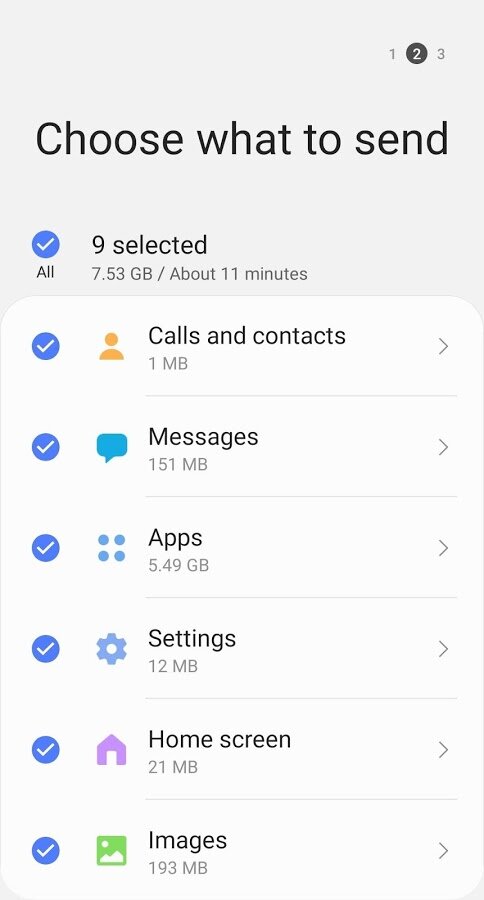The image is a detailed screenshot of a smartphone interface displaying a selection prompt titled "Choose what to send." Nine distinct data categories are highlighted, including Calls, Contacts, Messages, and Settings. It also shows multiple apps, with the total data size amounting to approximately 6.5 gigabytes. This extensive selection implies a potential data transfer, possibly to a cloud service for backup or migration purposes.